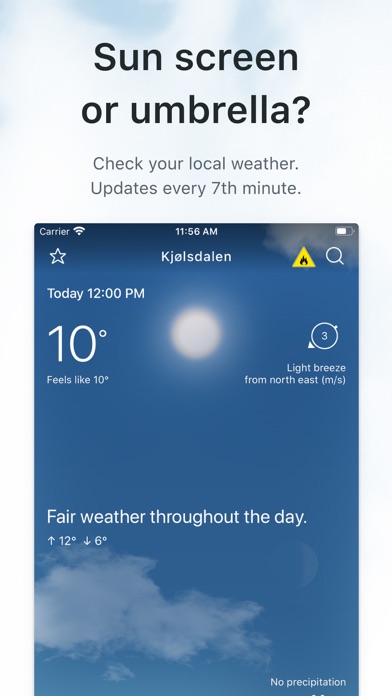The image appears to be a screenshot taken from a cell phone. The screenshot is a vertical rectangle featuring a weather update interface. The top third of the image has a light blue and white, sky-like background. Bold, black text stands out, displaying the message: "Sunscreen or umbrella? Check your local weather updates every seven minutes."

Below this header, the typical elements of a smartphone screen are visible— the time displayed as 11:56 in the middle, a battery symbol on the right, and a Wi-Fi symbol on the left. Directly under this information, a word in another language, "Kjeldalen," appears.

The main section of the image showcases a weather report against a backdrop of a blue sky with a single cloud in the bottom left corner and the sun positioned in the upper center. The weather details start with "Today, 12 PM" located in the upper left. Below this, it reads "10 degrees, feels like 10 degrees." The phrase "Fair weather throughout the day" is visible above the cloud. 

In the upper right-hand corner, there's a circle with an arrow and the number 3 inside it, indicating a "light breeze from the northeast." Finally, in the bottom right corner, it states "No precipitation."